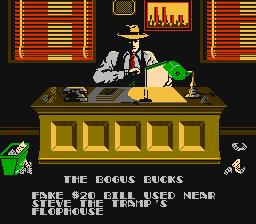The image depicts a computer-rendered, two-dimensional scene of a human figure seated at a large yellow wooden desk. The desk features decorative elements, specifically five raised sections on its front. Positioned atop the desk are a silver and green desk lamp, a black telephone, and several brown books. The desk surface appears to be brown.

The figure sitting at the desk wears a large-brimmed yellow hat, a white shirt, a red tie, and a blue or dark-colored vest. Behind the figure, there are horizontal red and yellow window blinds that are closed. Also visible is a framed picture with red and yellow elements. The rest of the background is predominantly black. To the side of the desk, there is a green waste bin overflowing with what appears to be white and black papers and other items.